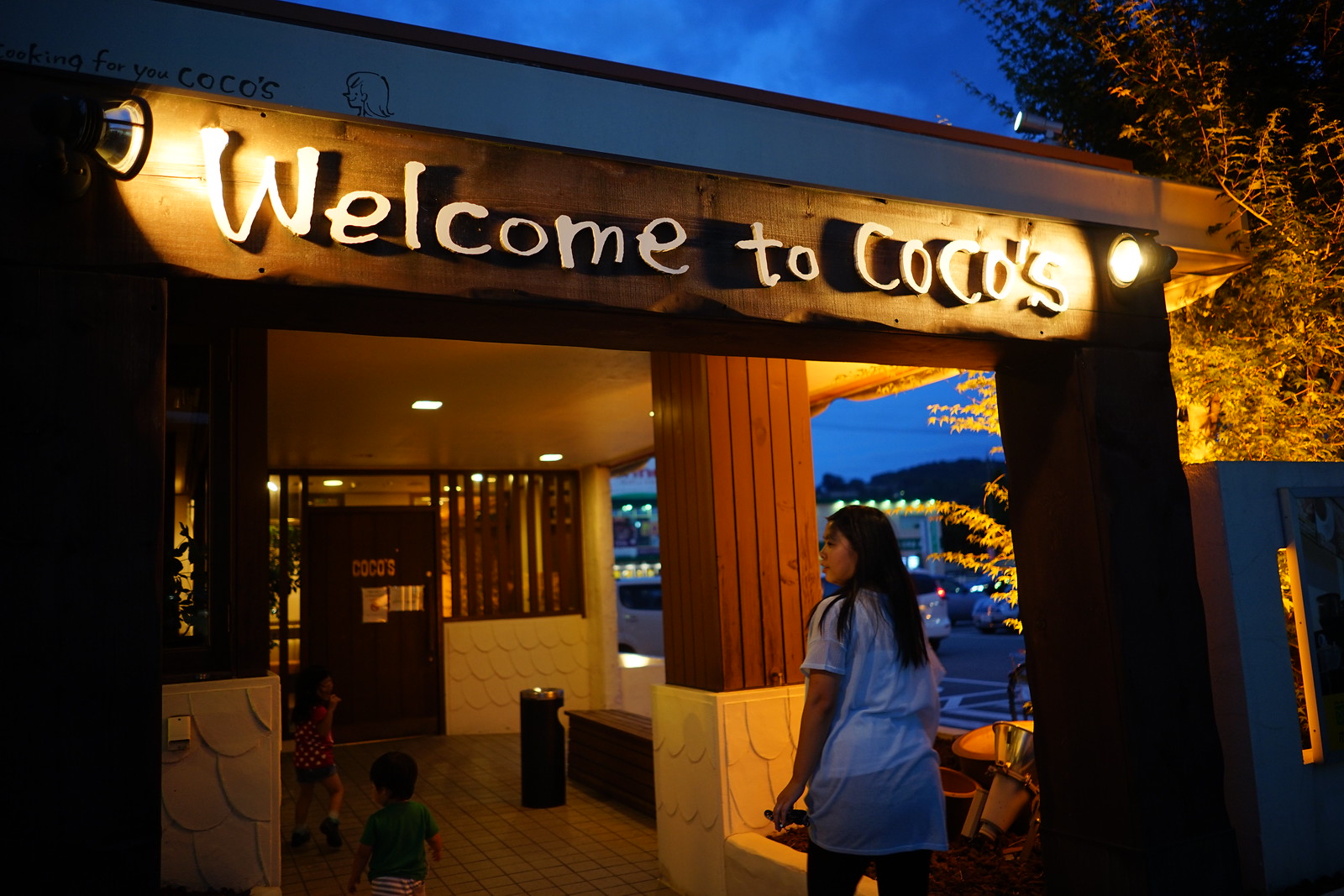In this evocative photograph captured during an overcast twilight evening, a woman with dark hair, dressed in a long gray shirt, walks toward the warmly lit entrance of a restaurant named Coco's. The entrance is adorned with a wooden sign illuminated by flashing lights that read, "Welcome to Coco's." The scene features a tile-floored foyer entryway with visible pillars and a trash can, leading to the main door. In the background, the soft twilight blue sky contrasts against the subdued lighting of other establishments and twinkling lights scattered among the trees. The restaurant's interior appears invitingly brighter through the windows and above the doorway, casting a welcoming glow. Nearby, a couple of children are running towards the door, likely accompanied by the woman, enhancing the lively yet cozy ambiance of this evening snapshot.